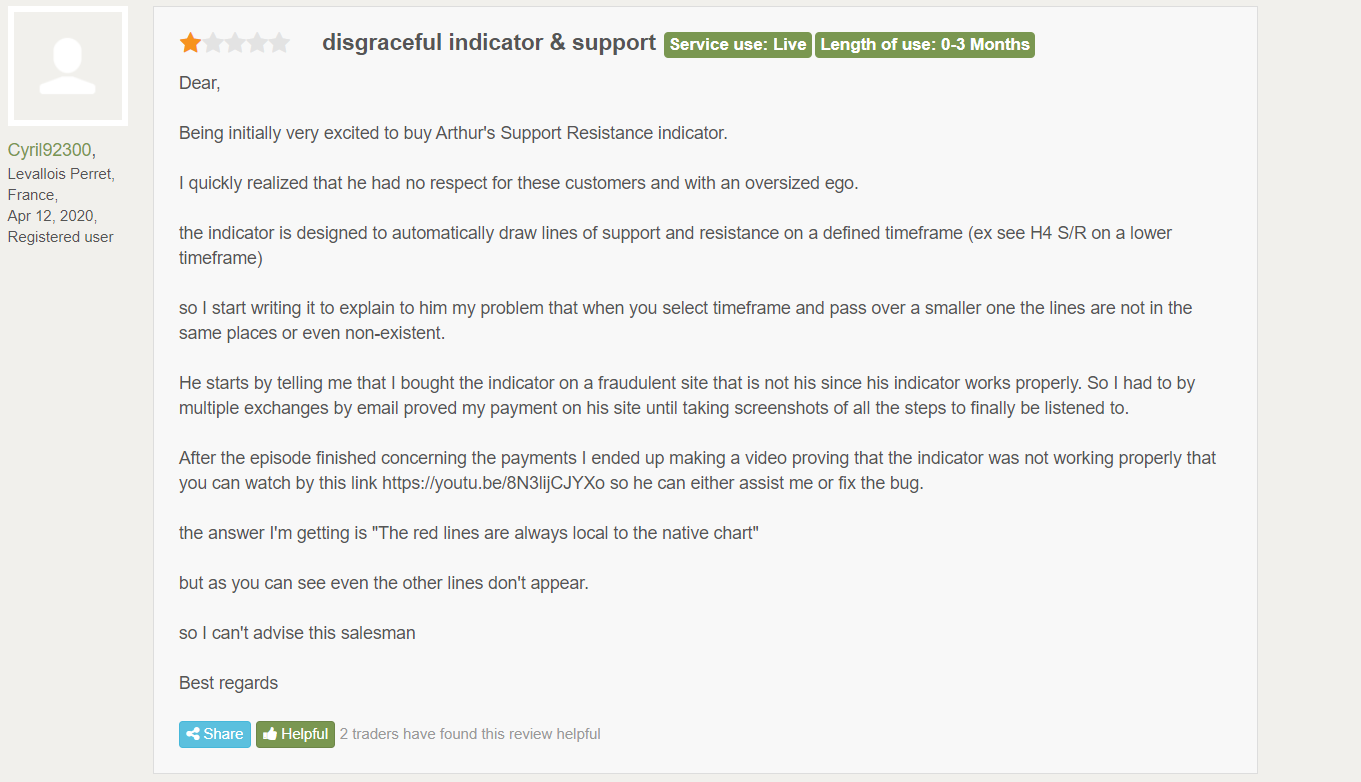Here is a cleaned-up and detailed caption for the image described:

---

**Review Screenshot Detailing Poor Customer Experience**

The image captures a screenshot of a customer review on a computer screen. It's notable that the left side features a gray vertical band. In the upper left corner of the screen, there is a small square icon. Below this icon, the text reads: "CYRLL92300, Lévi-Hauss-Perret, France, April 12, 2020, registered user."

To the right of this information, there is a larger light gray area containing the text of the review. At the top left of this section, there is a five-star rating scale with only the first star colored orange, indicating a one-star review. Next to the stars, the review headline states: "Disgraceful Indicator and Support." Below this, it notes: "Service Use: Live, Length of Use: 0-3 Months."

The review begins with a salutation "Dear," and proceeds to describe the customer's initial excitement about purchasing the "Authors Support Resistance Indicator," which quickly turned to disappointment. The customer criticizes the product's creator for having "no respect for these customers" and "an oversized ego." The review explains that the indicator is supposed to automatically draw lines of support and resistance on a defined time frame (referred to as XCH4S-R on a lower time frame).

The reviewer details their frustration with the indicator, noting that the lines don’t appear correctly when switching time frames. Despite contacting the creator to explain the issue, the customer was initially dismissed and told they had purchased the indicator from a fraudulent site. After a prolonged exchange of emails and proving their legitimate purchase through screenshots, the reviewer was finally listened to.

A video was created by the customer to demonstrate the malfunctioning indicator, which can be accessed via the provided link (https://youtu.be/n3lIJcJYXo). Despite this, the creator's reply was unsatisfactory, stating, "the red lines are always local to the native chart," which did not address the absence of other lines. The review concludes with the customer advising against this product and signing off with "Best regards."

---
This version provides a comprehensive and organized summary that fully captures the details and emotions conveyed in the original voice description.